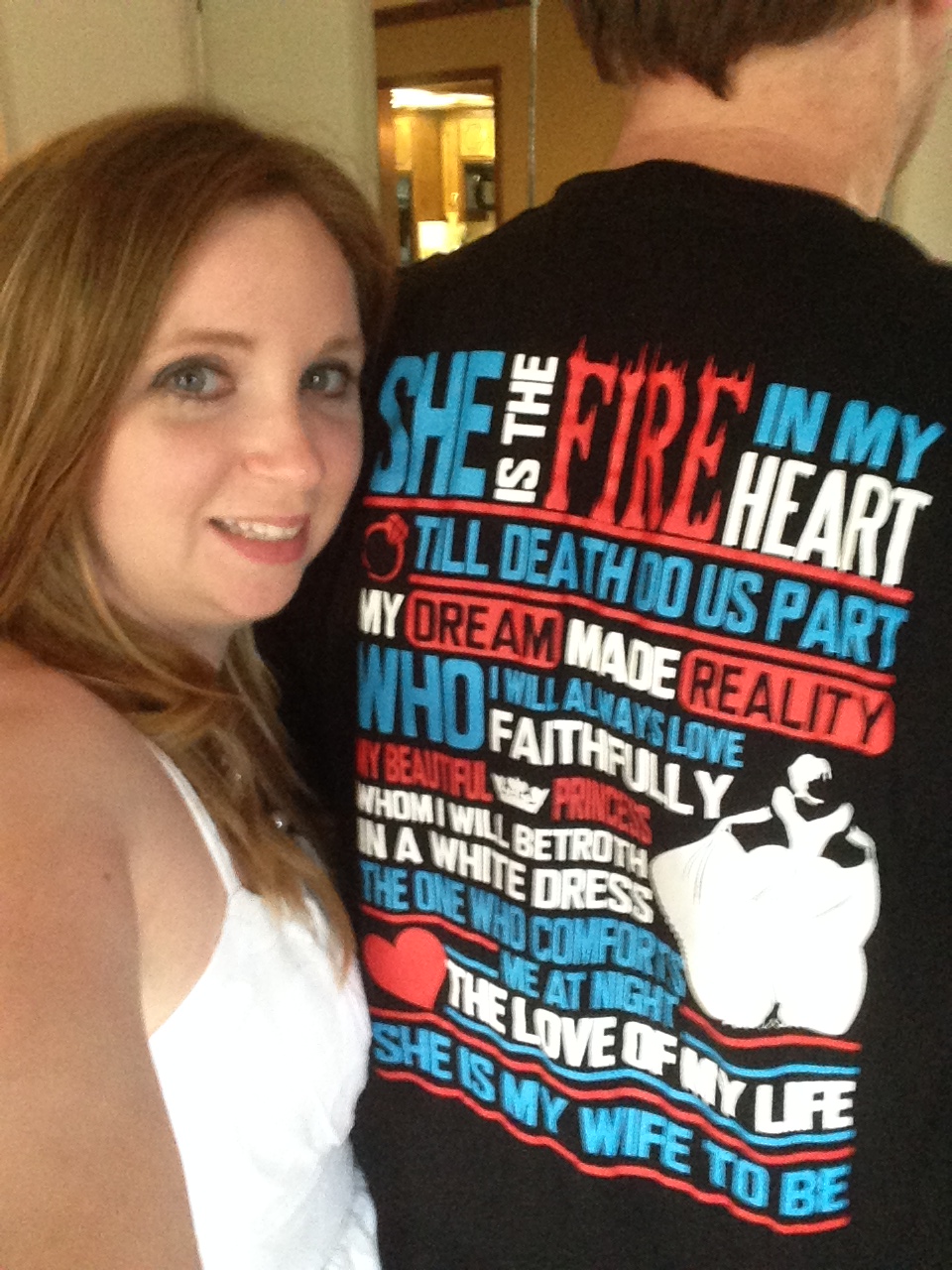The image shows a young woman pressed up against the back of a man, positioned to the left side of the frame. The young woman, likely under 20, has long brown hair, fair Caucasian skin, hazel eyes, and is wearing a white spaghetti strap tank top. She looks directly at the camera with a half-smile that conveys a mix of surprise and happiness. The man, whose back faces the camera, has short brown hair and wears a black shirt adorned with a paragraph of colorful text in blue, white, and red. The text on his shirt reads: "She is the fire in my heart till death do us part. My dream made reality. Who I will always love faithfully. My beautiful princess whom I will betroth in a white dress. The one who comforts me at night. The love of my life. She is my wife to be." The shirt also features various illustrations, including a woman holding a large dress, a heart, a princess crown, and a ring.